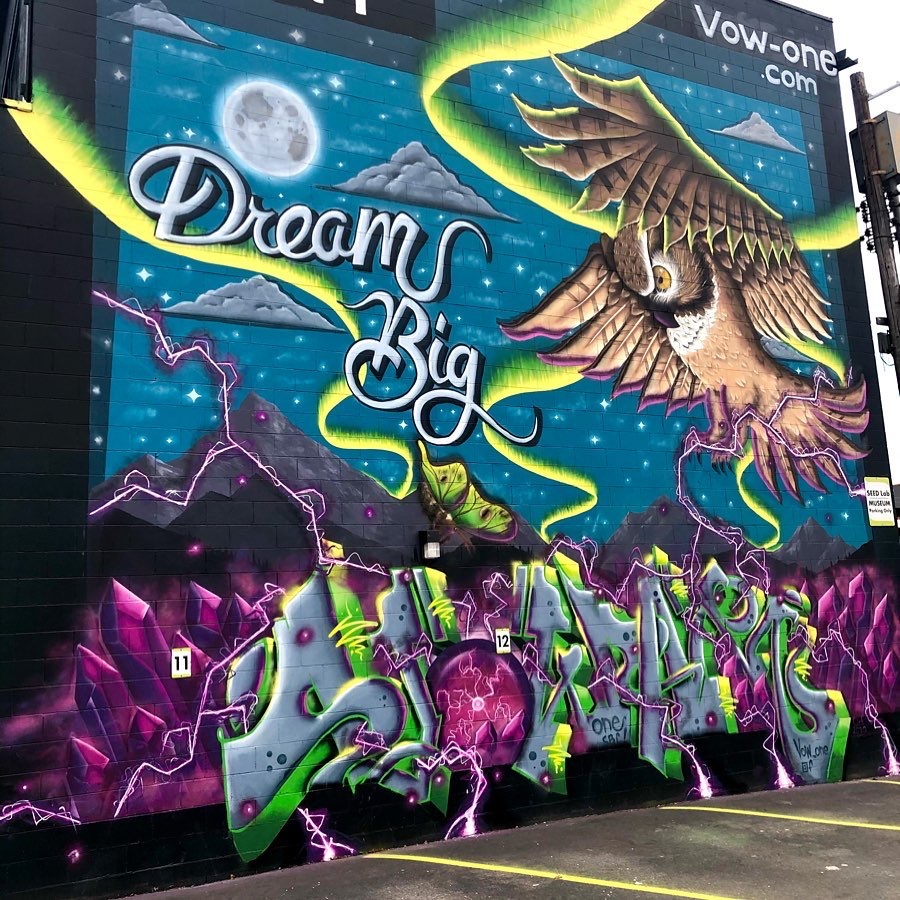The image showcases a large, detailed mural on a black brick wall adjacent to an asphalt parking lot with white painted lines visible at the bottom right corner. The mural intricately combines various elements against a backdrop of a blue sky adorned with white stars, a large, grey and white full moon in the upper left, and several grey clouds dispersed throughout. Prominent in the artwork is a majestic tan and dark brown owl with striking yellow eyes, positioned ominously on the right side, its wings dramatically spread and head tilted downward.

In the bottom portion of the mural, there are vibrant designs featuring purple diamond-like shapes protruding from the ground, interspersed with blue and grey graffiti-style letters that spell out an artist's name in an unreadable script. This area also contains a mystical purple orb emitting yellow and orange lightning bolts that stretch across the mural, adding an element of fantastical energy.

Additionally, a green butterfly can be seen fluttering within the scene, contributing to the whimsical and dream-like essence of the art. Hovering above everything, the inspirational phrase "Dream Big" is prominently displayed in white text, encapsulating the mural's imaginative spirit. The mural is a vibrant blend of natural and fantastical elements, creating an enchanting visual narrative that captures the viewer's imagination.